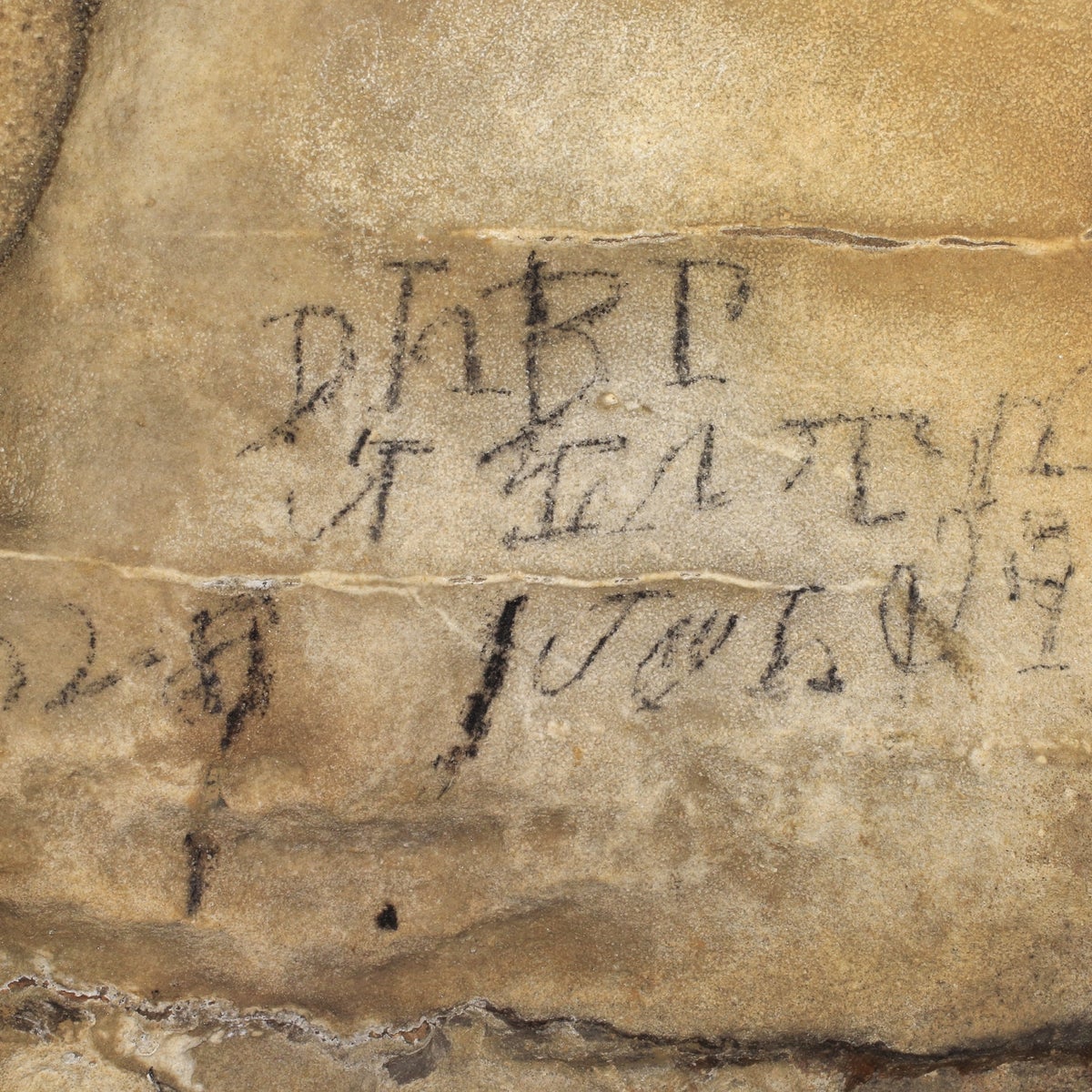The image appears to be a close-up photograph of an old, weathered stone or sidewalk surface. The surface is primarily light brown and sandy grey with various darker, grainy sections, indicative of aged stone. The stone is visibly cracked, with multiple fractures running through the center and top parts of the image. In the middle section of the surface, from left to right, are blurred, almost scribbled letters that appear to have been scratched or faded over time. The text is illegible for the most part, although some viewers believe they can faintly discern letters such as "D," "H," "B," and "P." The letters could have been written with something like chalk or black crayon. The texture of the surface suggests it could be stone or another rocky material, possibly even an old piece of fabric or animal skin with a granular, deteriorated texture.